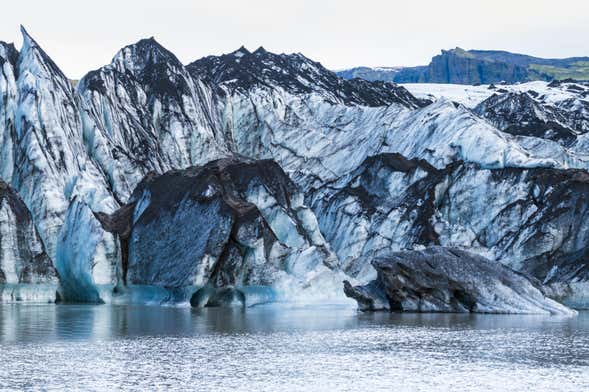The horizontally aligned rectangular painting showcases an outdoor scene dominated by glaciers and water, rendered in a primarily blue and white color palette. In the foreground lies a body of water displaying a mix of stillness and subtle ripples, the latter created by wind, giving parts of the water a white hue. The bottom right corner features a protrusion of a glacier dipping into the water. 

The mid-ground of the image is characterized by a vast expanse of white ice, with the glacier mountains rising up, their pointed tips a mixture of grey and white. These glaciers have prominent grey summits, indicating a rocky composition beneath the snow cover. 

In the background, another body of water stretches out under a grey sky, and a steep, barren cliff or mountain edge can be seen towards the top right corner. This distant mountain is primarily dark in color, devoid of snow, contrasting sharply against the lighter tones of the foreground glaciers. The overall clarity of the painting, paired with the atmospheric lighting, imparts a crisp and bright quality to the landscape. There's no text present in the image, keeping the viewer’s focus solely on the natural majesty of the glacial scene.